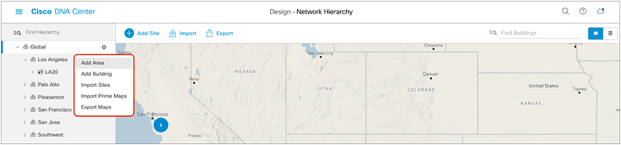The image displays a long rectangular interface in landscape orientation. At the top, there's a header with a white background. Centrally placed within the header, in black text, is the word "Design," followed by a bullet point, and then "Network Hierarchy" in bold black lettering. To the left, three blue lines indicate an expandable dropdown menu. In bold blue text, the word "Cisco" is visible, and to the right of it, "DNA Center" appears in blue, though not bold.

Below the header, a menu with a light gray background and gray text is visible. The first option, labeled "Find Hierarchy," features a bold gray magnifying glass icon to its left. Beneath this, the word "Global" is displayed, and the dropdown menu is expanded. "Los Angeles" is listed underneath, and to its right, an overlay area is highlighted with a red rounded square border. The selected option, "Add area," stands out against the light gray background. 

Additional options listed below "Los Angeles" include "Add Building," "Import Sites," "Import Prime Maps," and "Export Maps." Next, a building identifier labeled "LA 20" in capital letters is noted. Following this, "Palo Alto" is visible, while the subsequent entry is partially obscured. The list then continues with "San Francisco," "San Jose," and "Southwest."

Towards the bottom, there are three blue options. The first displays a blue circle with a white plus sign at its center, labeled "Add Site." The second option presents a share button icon, represented by a rectangle with a blue outline and a right-pointing arrow, labeled "Import." The third option, featuring the same icon, but with an arrow pointing up, is labeled "Export."